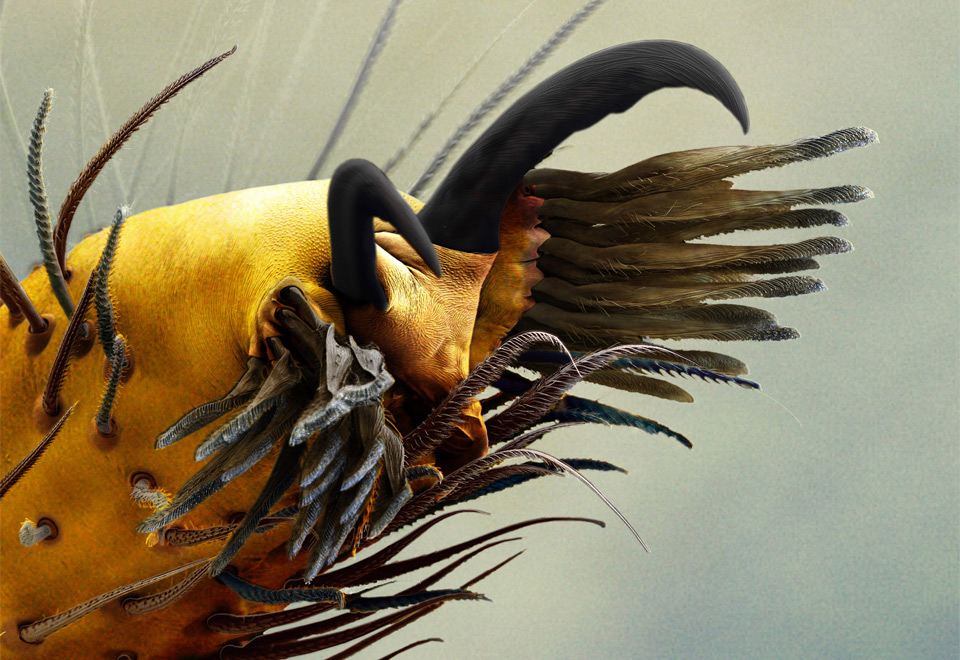In this highly detailed, microscopic-style photograph against a gray background, the viewer's attention is drawn to an unusual, organic structure occupying the majority of the frame. On the left side, emerging from the bottom and extending towards the center of the image, is a yellowish, leathery body that hints at a fabric-like texture. This central form suggests an almost alien or underwater creature, captivating with its distinct appearance.

Protruding from this yellowish shell are numerous tentacle-like extensions. At the top, several short, fuzzy hairs or tentacles rise upwards, giving a wispy texture to the top of this entity. On the right side, a multitude of longer, gray and black tentacles splay outwards, adding to the complex, spiny aesthetic of the organism. Additionally, there are two prominent, black horn-like structures protruding from the top of this body, which enhance its otherworldly appearance.

While the true nature of this entity remains ambiguous, it could be a microscopic view of an insect or a similarly scaled creature, with its intricate and highly detailed features creating a sense of wonder and intrigue.